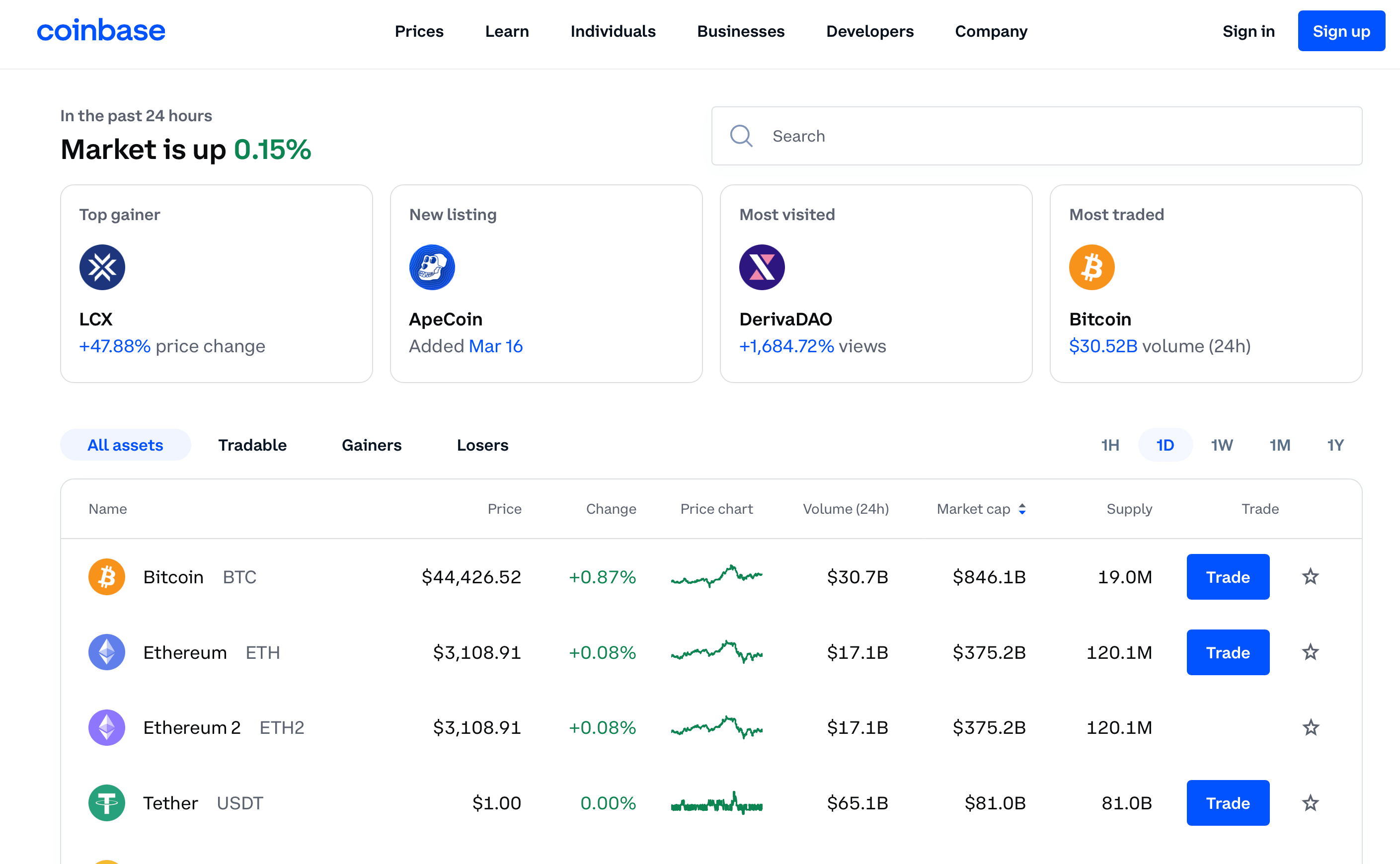The image depicts a predominantly white bathroom that prominently features a Coinbase webpage. At the top left-hand corner, the word "Coinbase" is displayed in blue. Below this, there is a navigation menu with tabs in black and blue labeled "Learn," "Prices," "Individuals," "Businesses," "Developers," "Company," and "Sign-in." To the right of this menu is a blue rectangle with white text that reads "Sign-up."

A thin gray line stretches across the page, segmenting it into sections. On the left side, there is an update reading "In the past 24 hours," followed by an indicator that the market is up by 0.15%, displayed in green.

Adjacent to this is a search box containing a gray magnifying glass icon and the text "Search" in gray. Below this are four rectangular boxes outlined in gray, each containing various pieces of information:

1. **Top Gainer:** 
    - LCX: +47.88% in blue, with the label "Price Change" in black.
2. **New Listing:**
    - ApeCoin added on March 16th, highlighted in blue.
3. **Most Visited:**
    - DerivaDAO: +1,684.72% in blue.
4. **Most Traded:**
    - Bitcoin: $30.52B in blue with "(24H)" in black.

Further down the page, the menu includes several tabs. The first tab, labeled "All Assets," is highlighted in blue, indicating the current view. Other tabs include "Tradeable," "Gainers," "Losers," "Bitcoin," "Ethereum," and "Theta," with a "Trade" button next to each cryptocurrency name.

The detailed webpage information overlaid onto the white bathroom wall creates a stark contrast, making the digital elements stand out prominently against the clean, monochromatic background.